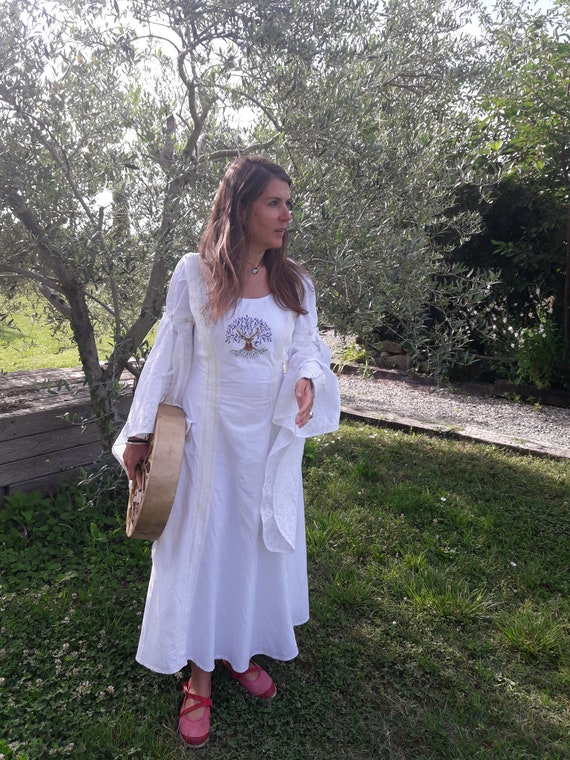In the center of this AI-generated image stands a woman who appears to be in a forest or backyard area. She is wearing a white sundress that features an intricate design: a purple tree with visible roots adorning the chest area. Her dress, paired with a shawl, displays subtle irregularities common in AI-generated images, such as extra fingers and abnormal clothing lines, which hint at its unnatural origin. She holds a gold-covered circular object in her right hand and wears pink and red ribboned shoes. The necklace she sports features a diamond stud pendant. The background reveals a light green tree, several bushes, and a wooden deck extending towards a gravel path, all under a bright, sunny sky. She is standing on short, green grass, adding to the lifelike yet slightly off-kilter scene.